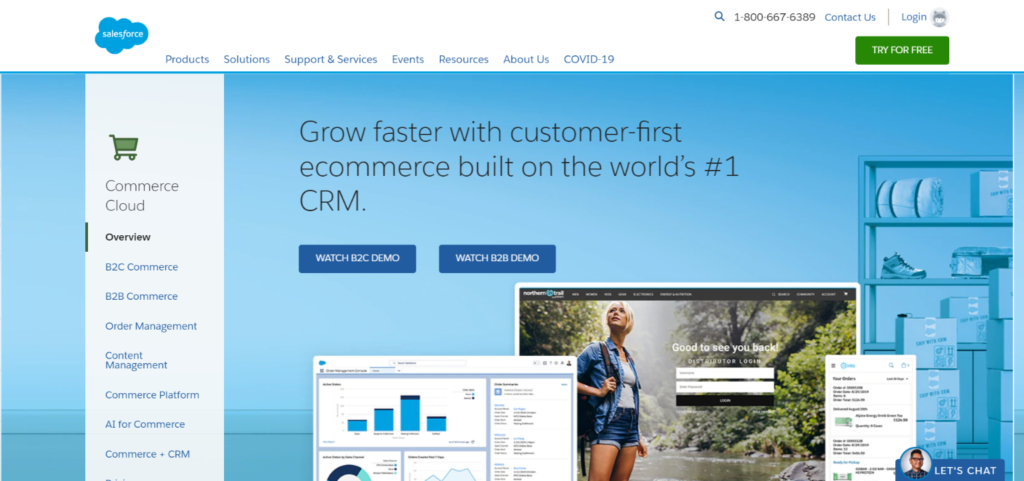The image depicts a detailed layout of an e-commerce support website, designed to facilitate online sales and customer relationship management. 

At the top, there's a solid white header featuring the Salesforce logo, accompanied by several navigation tabs labeled Products, Solutions, Support and Services, Events, Resources, About Us, and COVID-19. To the far right of the header, there is a magnifying glass icon for searching, a customer service number (1-800-667-6389), and options to Contact Us and Log In. A prominent "Try for Free" button is also visible.

The background features a shelf adorned with various items, including boxes, plates, and a shoe, suggesting an e-commerce context. On the website’s left side, there's a shopping cart icon with additional navigational options beneath it.

Centrally placed on the website is an impactful quote: "Grow faster with customer-first e-commerce built on the world's number one CRM." Below this quote are two call-to-action buttons labeled "Watch B2C Demo" and "Watch B2B Demo."

Towards the bottom of the screen, multiple graphical elements are displayed, including a bar graph, a circle graph, and a line graph, illustrating data analytics capabilities. Lastly, on the bottom right, there's an image of a woman gazing upwards, adding a human element to the website's design.